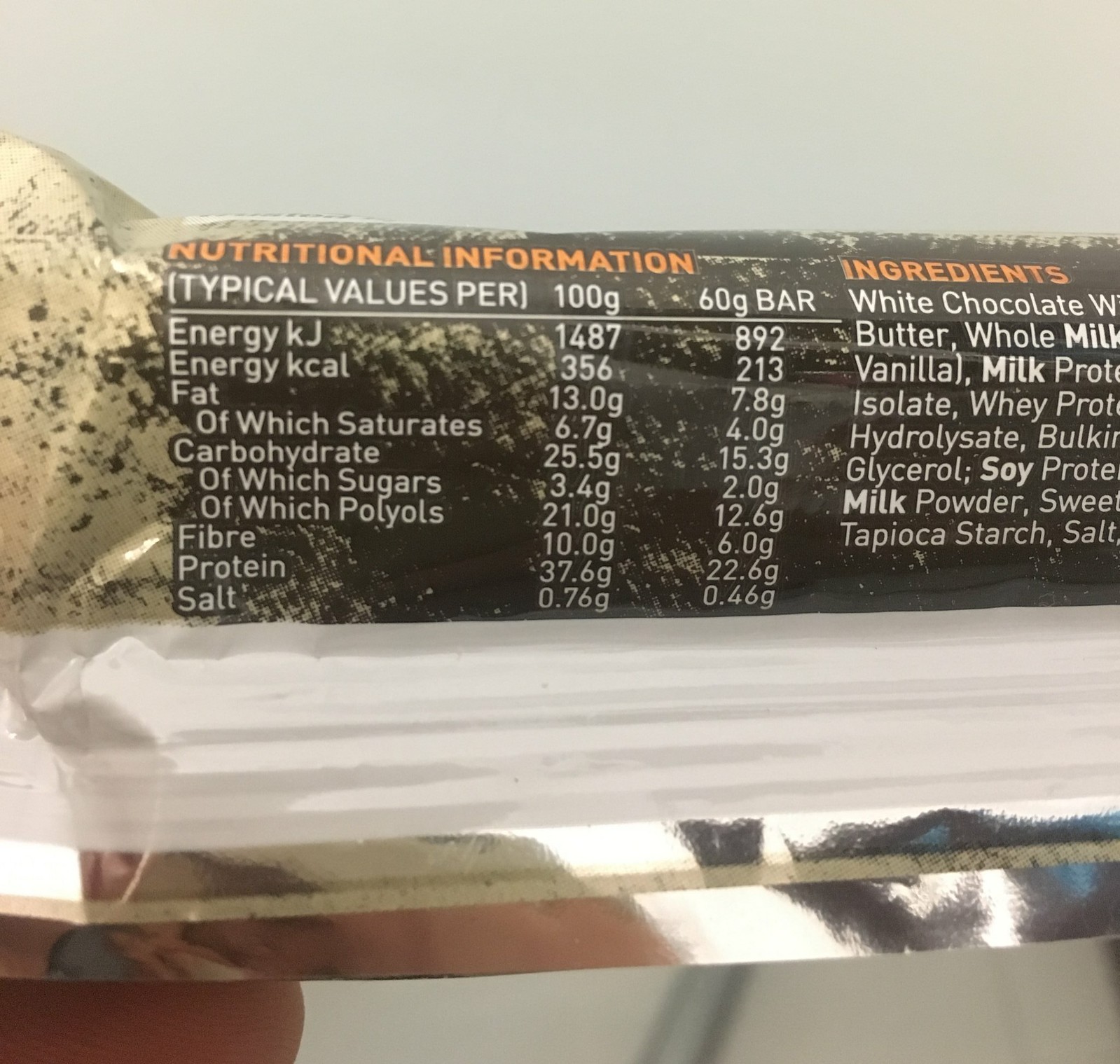This is a detailed photograph showcasing the nutritional information and ingredients of a powder mix, likely a protein powder, as inferred from the nutritional values displayed. In bold orange font at the top, the label reads "Nutritional Information." Below, in white font, it details "Typical values per 100 grams or a 60-gram bar." The nutritional breakdown reveals the energy content as 1487 kJ per 100 grams and 892 kJ per 60-gram bar. The calorie count follows, indicating 356 kcal per 100 grams and 213 kcal per 60-gram bar. The fat content is listed as 13 grams per 100 grams and 7.8 grams per 60-gram bar. Continuing through the nutritional facts, it shows the carbohydrate, fiber, protein, and salt content meticulously detailed. On the right side of the package, the ingredients are clearly listed, including white chocolate, whole milk, butter, and milk powder.